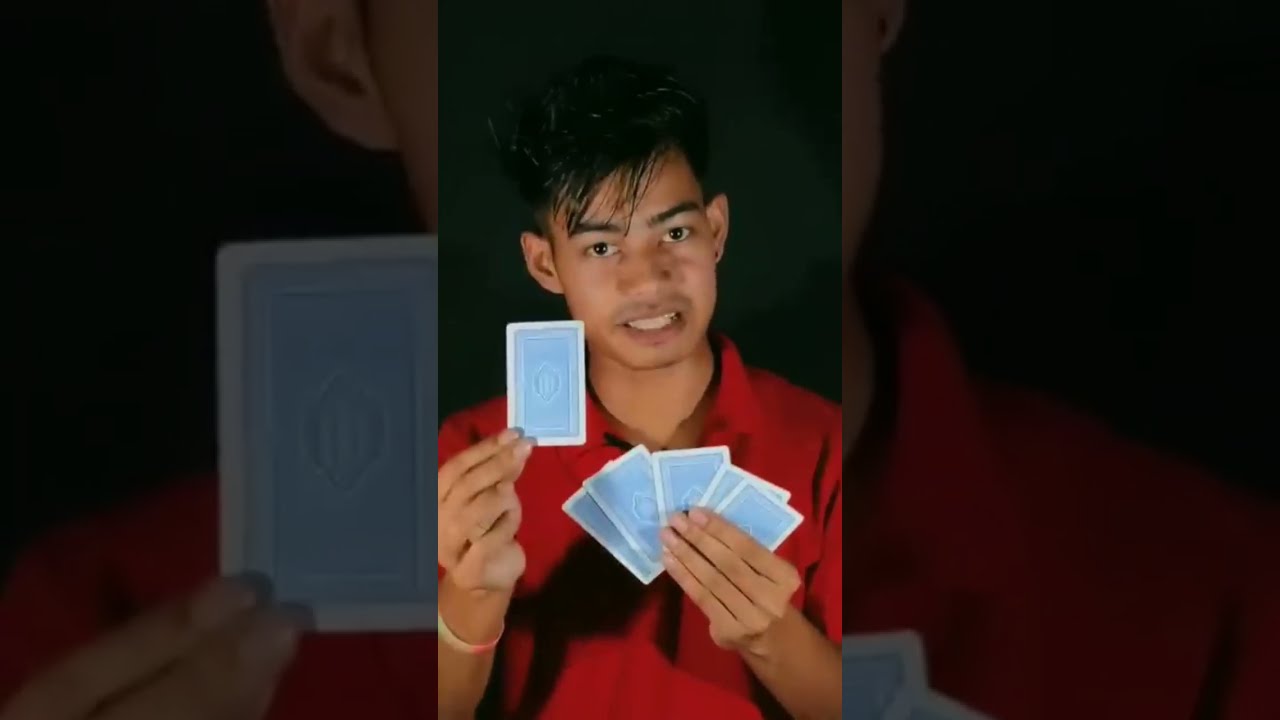The image appears to be a screenshot captured from a vertical video, likely from a social media platform such as TikTok or Instagram. The central third of the image showcases a photorealistic depiction of a young Asian man, perhaps in his early 20s, with dark skin, black hair falling over his forehead, dark eyebrows, and expressive dark eyes. His mouth is open, showing his teeth as if he is speaking or explaining something with an intense look on his face. He is wearing a red collared T-shirt and a red and green bracelet on his left wrist. In his right hand, he is holding a fanned-out set of five playing cards with blue designs on the back, while his left hand holds a single card above the rest. The background is dark green, and the outer thirds of the image feature zoomed-in and darkened portions of the same photograph, creating an emphasis on the central subject.